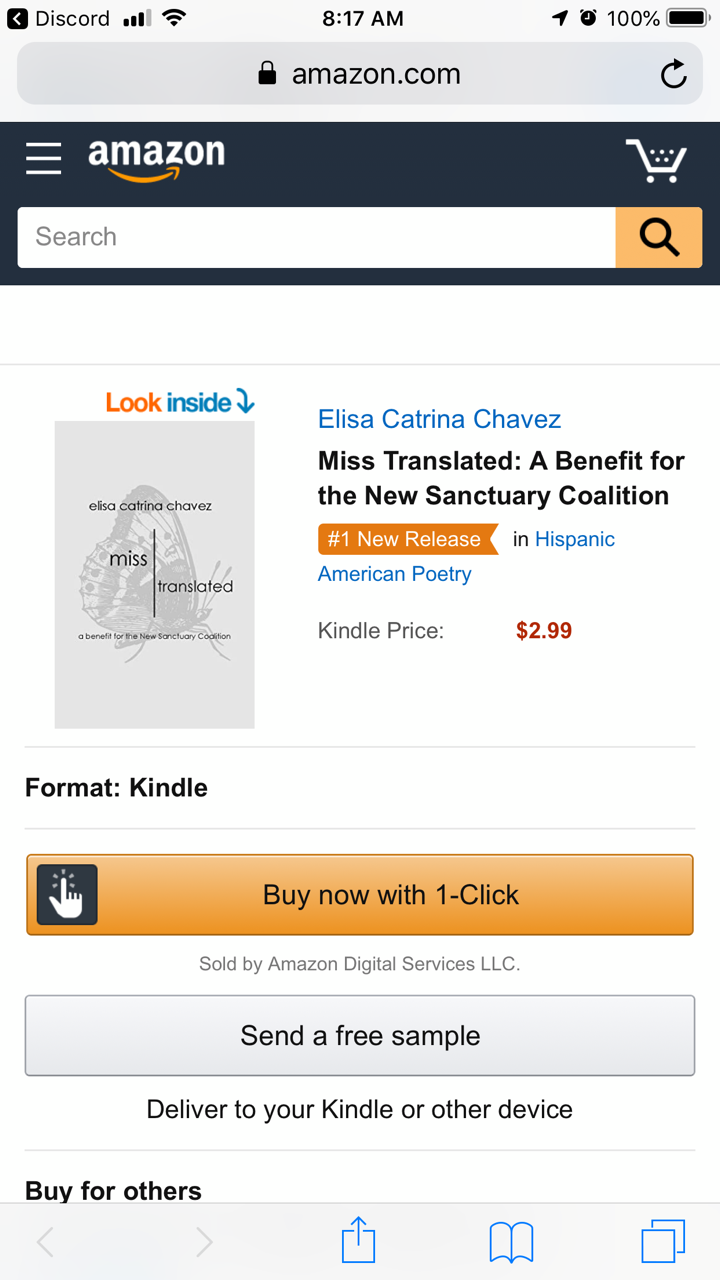This is a screenshot of an Amazon webpage displaying a product listing for the book titled "Mistranslated," which supports the New Sanctuary Coalition. Notably, it is designated as the number one new release in the category of Hispanic American Poetry, as indicated by the prominent orange "New Release" tag. The Kindle edition of the book is priced at $2.99, emphasized in bold red numbers.

To the left of the pricing information, there is an image of the book cover, featuring a butterfly in the background. The author's name is positioned at the top, with the book title prominently displayed in the center. Beneath the title, the subtitle is visible, and there is a "Look Inside" button that allows potential buyers to preview the book's content.

Further down, the format is specified as Kindle, with no alternative formats available. The page also features an orange "Buy now with 1-Click" button, accompanied by a cart icon to its left. Below this, the listing indicates that the book is sold by Amazon Digital Services, LLC. Additionally, there is an option to send a free sample of the book.